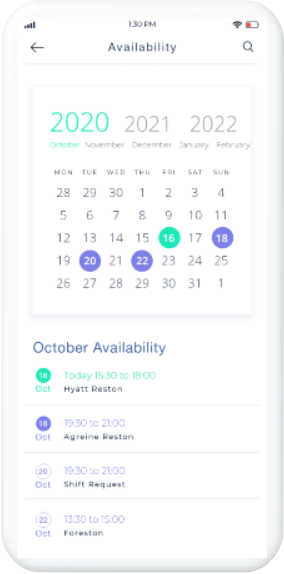This is a detailed screenshot of a smartphone displaying its calendar application. At the top of the screen, the status indicators show a full signal strength with all four bars, the time being 1:30 PM, a connected Wi-Fi signal, and a nearly depleted battery shown in red, likely below 20%.

Beneath these indicators, the calendar function interface is visible. The display highlights the years 2020, 2021, and 2022, with the year 2020 prominently selected. The month October is also highlighted. Specific dates within October are marked with different colored circles: October 16th is circled in green, while October 18th, 20th, and 22nd are circled in purple.

Further below, the section titled "October Availability" lists detailed event entries for the selected dates. The entry for "October 16" states "Today," with the timeframe 15:30 - 18:00 and the location "Hyatt, Reston." The entry for "October 18" shows "1930 - 2100," followed by the name "Arjean, Resters." For "October 20," the time "1930 - 2100" is marked, with the note "Shift request." Lastly, the entry for "October 22" lists the time "1330 - 1500" with a note that appears to read "Forestation."